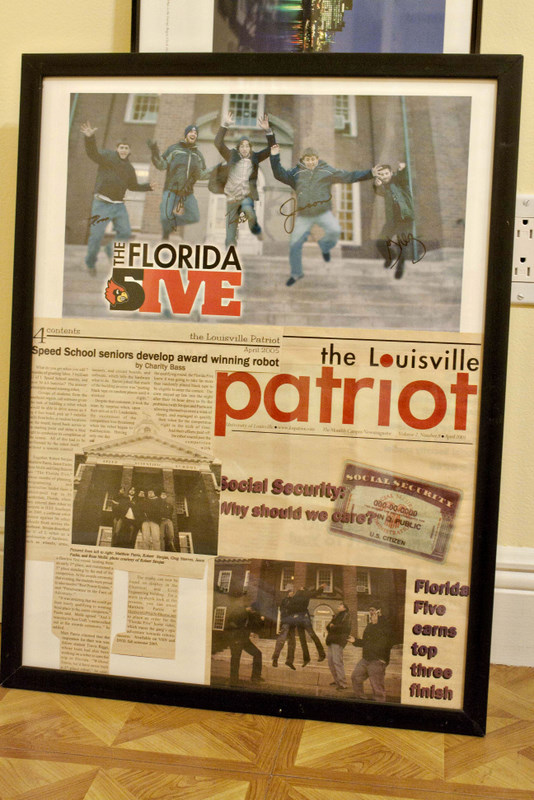The image showcases a framed collection of yellowed newspaper clippings from the early 2000s, leaning against a wall. Dominating the frame is a photograph of five high school boys, mid-air as they leap off a staircase in jubilant celebration. Above them, a prominent logo reads "Florida Cardinal Five," indicating their recognition. The various clippings include headlines such as "Speed School Seniors Developed Award-Winning Robot," highlighting the group's impressive achievement. Another notable detail is an image of a Social Security card accompanied by the question, "Why Should We Care?" further emphasizing the significance of their accomplishments. Additionally, a header proudly announces, "Florida Five Earns Top Three Finishes," tying the boys' exuberant display to their recent successes in their endeavors.